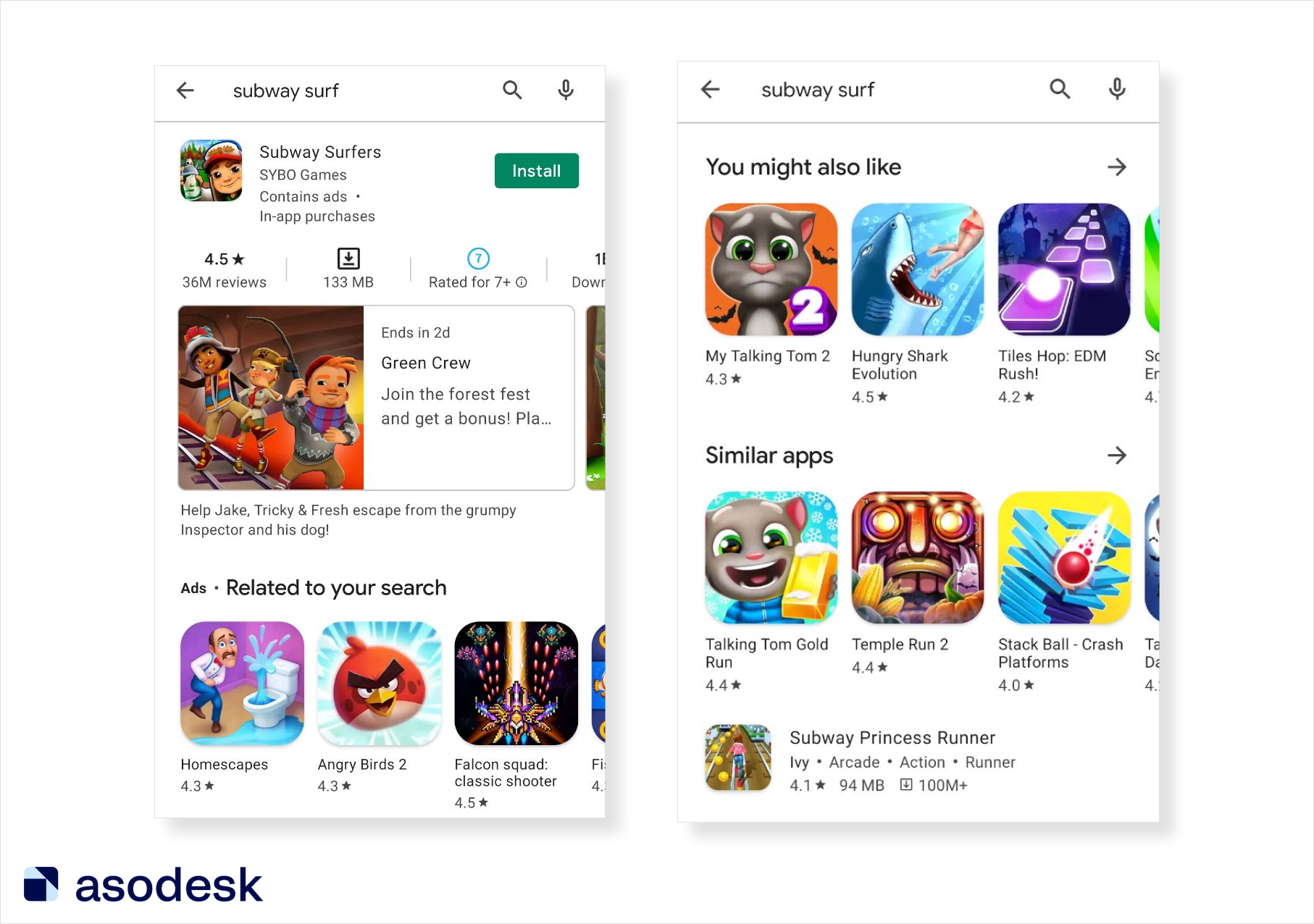This image consists of two screenshots, presumably from an app store, most likely the Google Play Store, given the layout and features. Both screenshots prominently feature the search term "Subway Surf" in the search bar at the top.

**Left Screenshot:**
- A highlighted game, "Subway Surfers," is displayed with a recognizable icon featuring a character wearing a hat with beige skin. 
- A green "Install" button is positioned to the right of the game icon.
- Additional details include a rating of 4.5 stars based on 36 million reviews, the app size of 130 megabytes, and an age rating of 7+.
- Beneath the game details, a promotional banner indicates an ongoing event named "Forest Fest," which ends in two days, offering a bonus.
- Below the promotion, there is an advertisement section featuring games related to "Subway Surfers" such as Homescapes, Angry Birds 2, and Falcon Squad.

**Right Screenshot:**
- Positioned below the game search results is a "You might also like" section, suggesting various apps. These include My Talking Tom 2 (showcasing a cat on an orange background), Hungry Shark Evolution (featuring a shark chasing a woman in a red bikini), Tileshop (EDM Rush) (depicting purple tiles receding into the distance at an angle).
- Under this section is a list of "Similar apps," featuring multiple applications such as Talking Tom Gold Run, Temple Run 2, Stack Ball, Crash Platforms, and Subway Princess Runner.
- In the bottom left of this screenshot, there is a modern minimalist logo alongside the words "ASO Desk."

The comprehensive visual and textual information provided creates a detailed view of how app recommendations and promotions might appear within the Google Play Store environment.